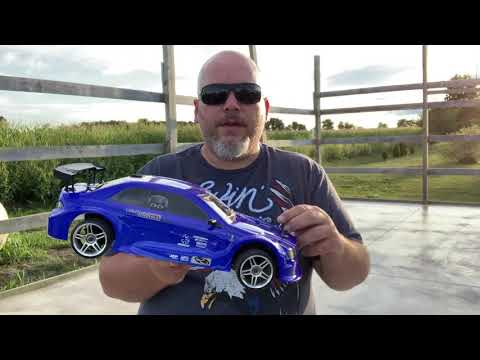In the image, a heavyset, bald Caucasian man with a gray beard and mustache is showcased standing outdoors. He sports black sunglasses and a gray short sleeve shirt, possibly featuring a bald eagle design partially covered by the item in his hand. He stands on a cement platform surrounded by what appears to be a wooden fence. In his hand, he holds a medium-sized, royal blue model sports car adorned with silver custom wheels and a black spoiler. Although the car displays some text and a number, these details are not clearly readable. Behind the man, the scene extends to a vibrant green landscape, including tall grasses, rows of crops that appear to be cornfields, and clusters of leafy trees. The sky above is mostly white with some visible clouds, suggesting an overcast day.